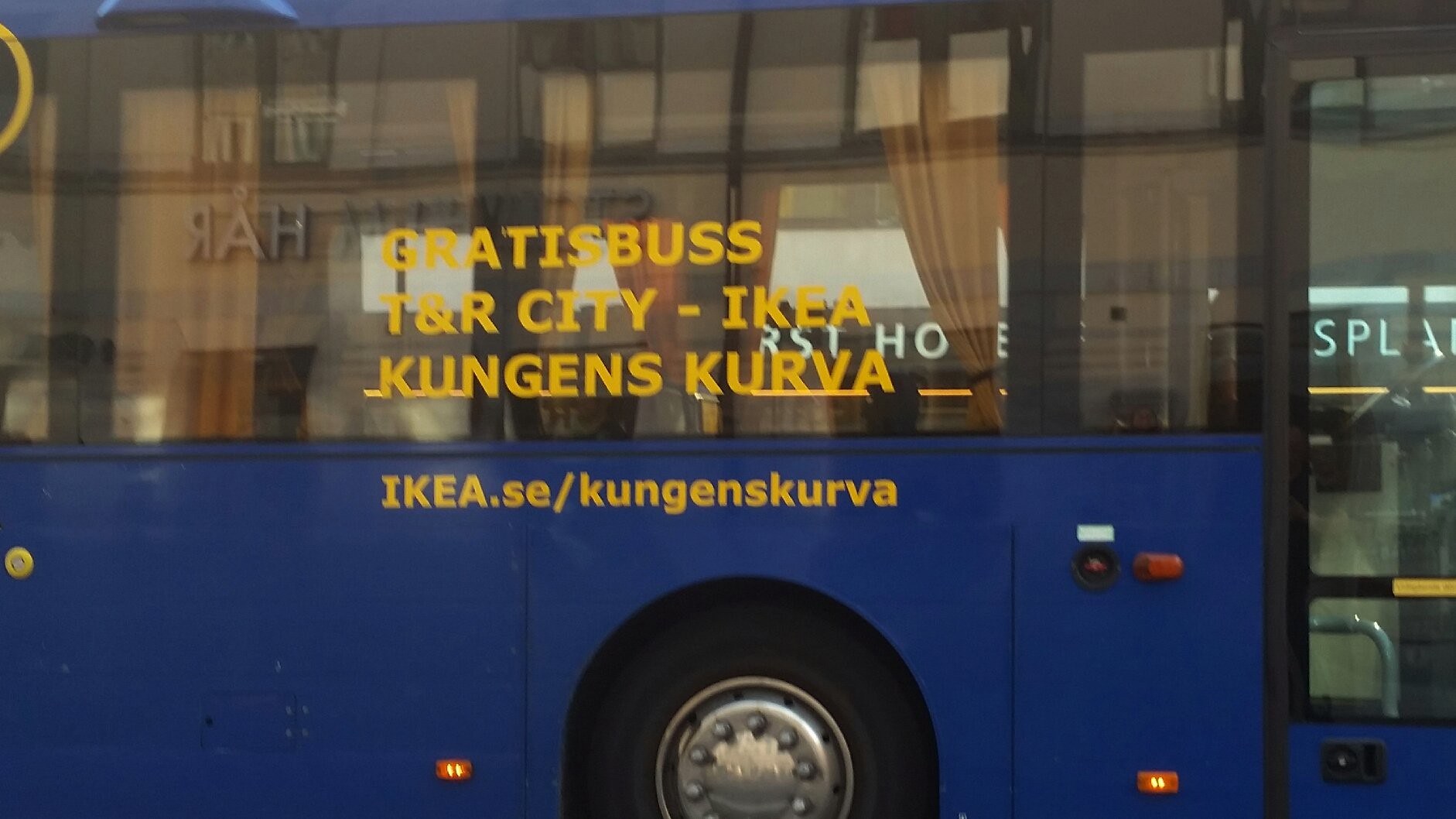This outdoor photograph showcases the side of a striking IKEA city bus, journeying from right to left in the frame. Dominating the foreground, the bus flaunts its vivid dark blue lower half with prominent glass windows above. Through these windows, reflections of a nearby building's curtains are visible, along with the backward letters "HAR." The bus itself is adorned with clear, bold yellow lettering that proclaims "GRATIS BUSS" and "TNR City - IKEA," followed by "Kungens Kurva," indicating its route. Just below this text, an additional line reads "IKEA.se/KungensKurva." Details like black wheels, safety lights, and partially visible bus doors with sleek handles underscore the practicality of this free transit service, seemingly provided for IKEA shoppers. The rear portion of the bus hints at its parked or operational status with some lights on, indicating readiness for its next journey.